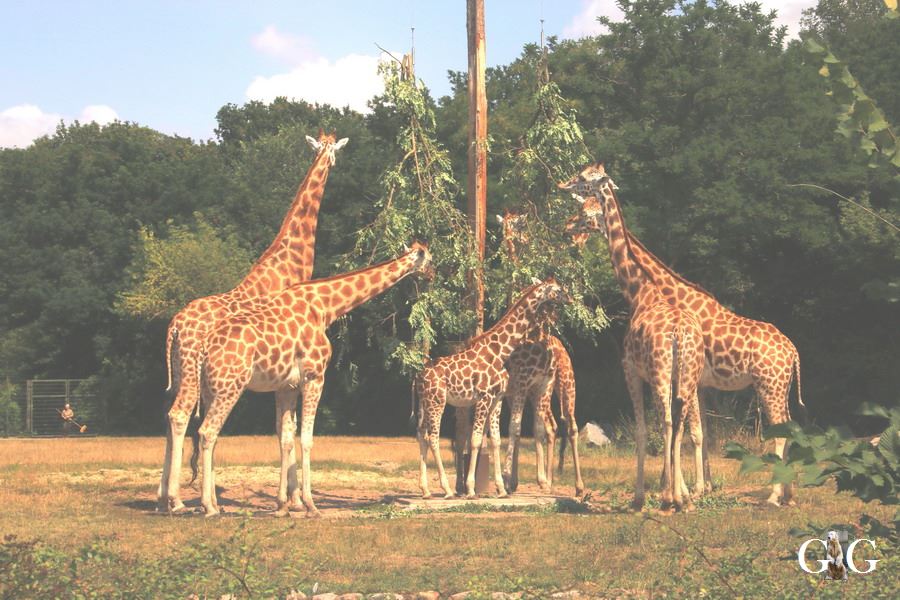The photograph appears to be a vintage, colorized image, possibly from the 1970s to early 1990s. It showcases six giraffes, some of which are adults while others appear to be juveniles, gathered around a tall utility pole in a zoo habitat. This pole is centrally located in the image and has branches hung from it, mimicking a tree and allowing the giraffes to feed on the suspended foliage. The background features a forest with tall trees, a blue sky with billowing white clouds, and a dry grassy plain consisting of mixed brown and green short grass. In the bottom left corner, a tall wire gate fence, typical of zoo enclosures, is visible with a small human figure standing in front, holding a broom. The person, dressed in a light-colored shirt, underscores the zoo setting of the habitat. In the bottom right corner of the image, there's a logo comprising two capital G's with a polar bear standing on its hind legs positioned between them, serving as an identifier for the content creator.